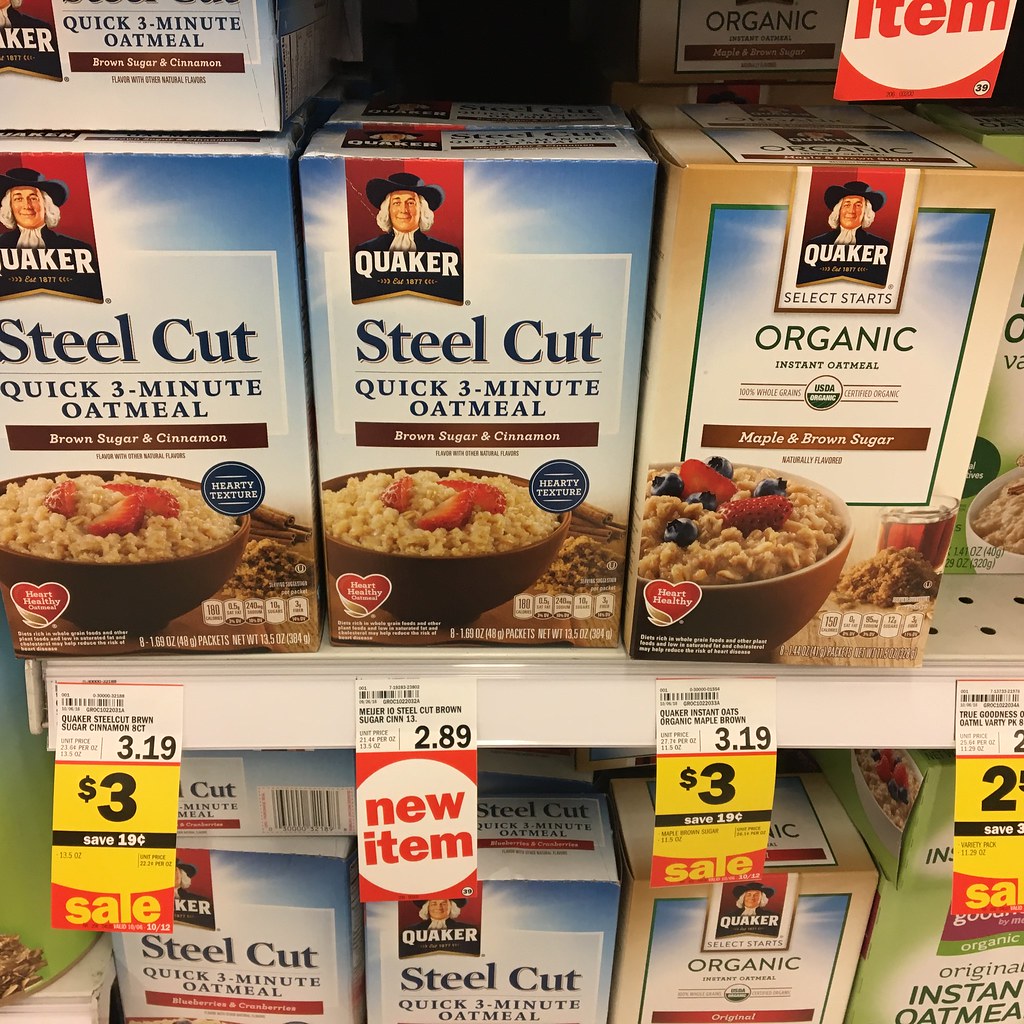This image captures a neatly arranged display of Quaker oatmeal boxes on two supermarket shelves. The featured brand, Quaker, is easily recognizable by its iconic logo of the Quaker man donning a black hat and white wig, with the word "Quaker" prominently displayed. 

On the top shelf, rows of steel-cut quick three-minute oatmeal are encased in blue boxes. Each box showcases an appetizing image of a brown bowl filled with oatmeal, garnished with fresh strawberries. Adjacent to these, an organic variety stands out in beige packaging, featuring a similar bowl of oatmeal, adorned with strawberries and blueberries on the left side.

The bottom shelf also houses additional steel-cut quick three-minute oatmeal boxes. Price tags, including a noticeable yellow tag indicating a discount, reveal that the steel-cut oatmeal is priced at three dollars, adding a touch of practical information for prospective shoppers.